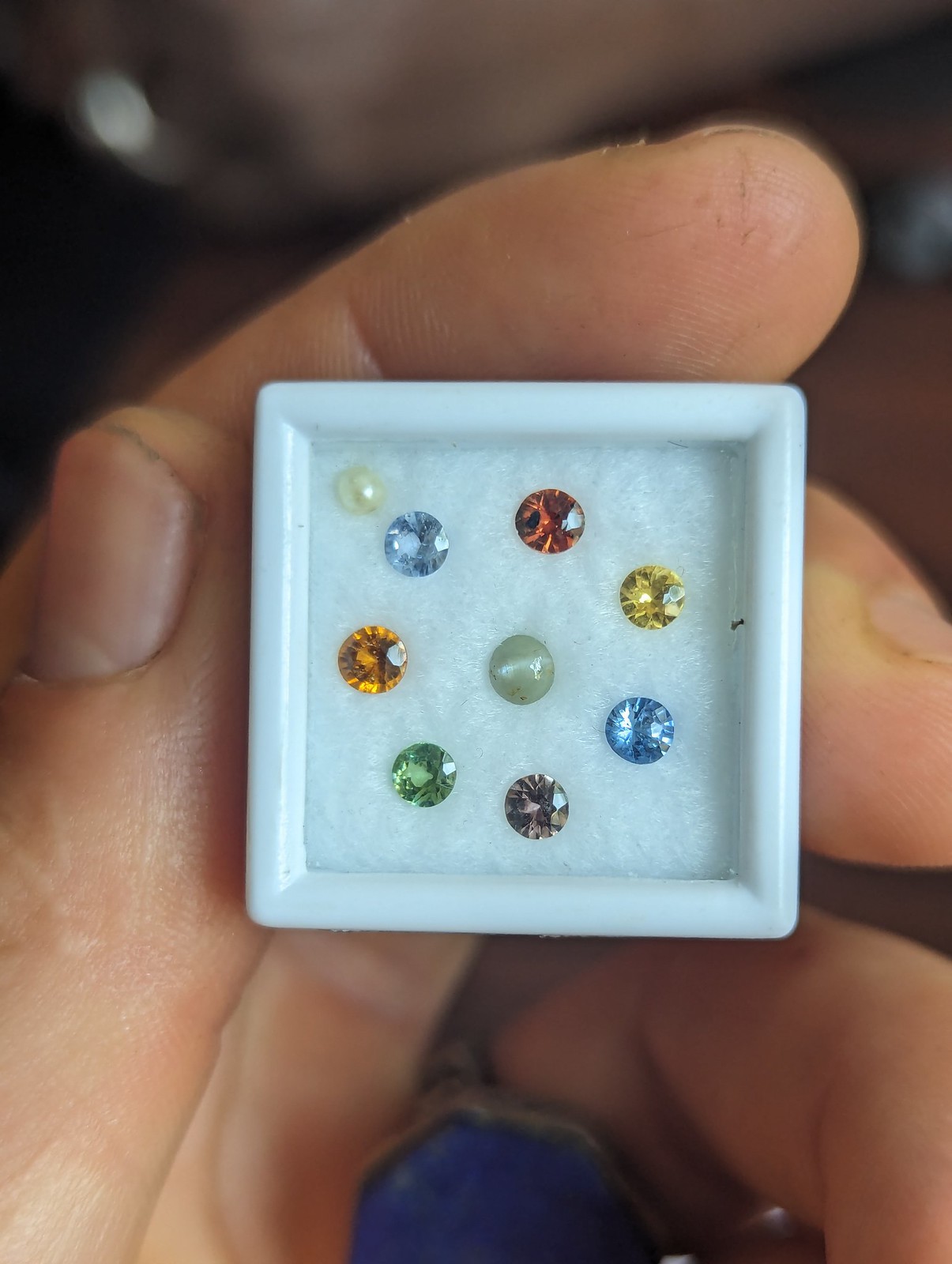In this detailed photo, we observe a tan-skinned hand, possibly of a man, holding a small white square that resembles porcelain. This white square contains a soft layer, likely cotton, on which various colored gemstones and pearls are meticulously arranged. The gemstones, presented in a circular pattern, shine brilliantly with multiple cuts and bezels, reflecting light from their polished surfaces. The circle includes a variety of stones: a red, orange, yellow, blue, green, and dark (black or brown) gemstone, all radiating in a clockwise sequence. At the center of this circle is a darker gray gemstone, resembling a pearl, while a smaller white pearl rests in the top left-hand corner of the box. The hand holding this jewelry exhibits signs of hard work, with visible small cuts, scuff marks, and dirty fingernails on the short thumb, index, and middle fingers. The background is blurred, drawing complete focus to the intricate details of the hand and the treasured contents of the white square.